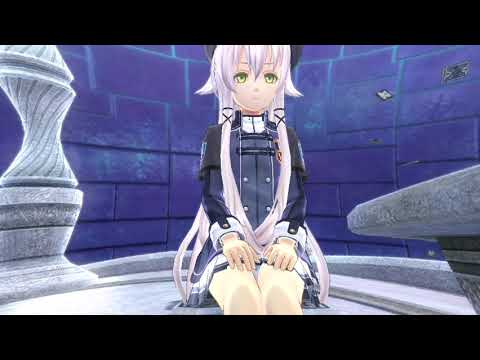This image portrays a young anime girl with grayish-purple hair and large, expressive green eyes. Her hair has distinctive strands that curl up on either side. The girl is sitting down on a gray cement floor with her back straight and her legs closed together. She wears a dark blue jacket-like top, adorned with four white buttons and two horizontal dark blue lines near her neck. Her hands rest delicately on her thighs. The jacket's long sleeves feature darker blue outlines running down the arms. A blue skirt dress completes her attire. She has a stoic, solemn expression, staring straight ahead without a smile or frown. The background consists of large blue bricks or tiles, some shaped like rectangles and others forming L-shapes, creating a geometric pattern. Despite the cement structures around her, including potential benches, the focus remains on her serene, solitary presence against the vividly detailed backdrop.